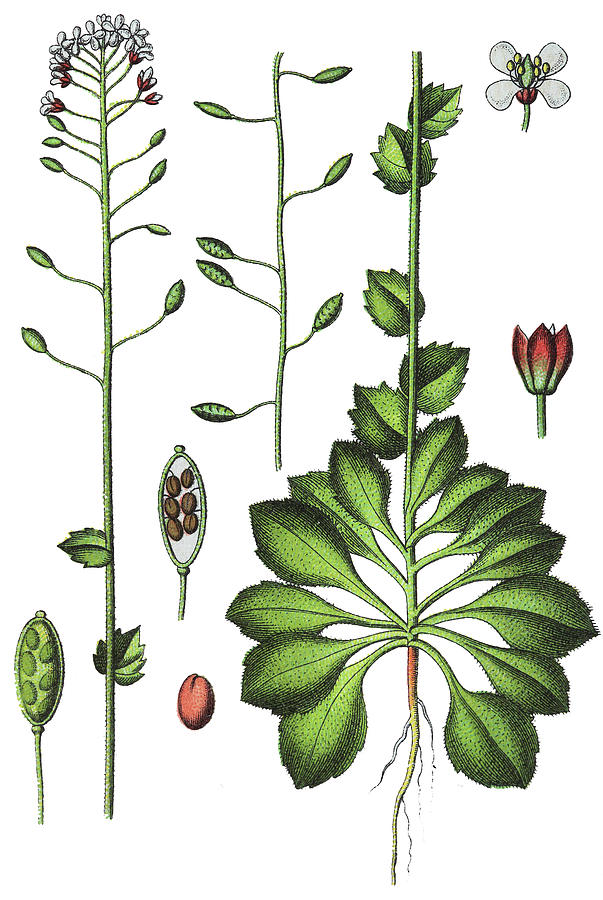This illustration-style image features a vibrant collection of green leafy plants, some of which exhibit a distinctive black shadowing effect. Among them, you can see various white and red flowering plants interspersed with green flower buds. The red and green petals of some flowers display a slight curl, adding to their intricate detail. Set against a white background, the image has an artistic, grainy texture that enhances its visual appeal. A very tall green plant prominently stands out with its red and white blossoms, while shorter plants and isolated flower heads contribute to the overall composition. Notably, one plant at the bottom showcases visible roots with a yellow and white hue, adding an element of realism. The entire scene is imbued with a fuzzy, almost dreamlike quality, making it a captivating and detailed portrayal of flora.